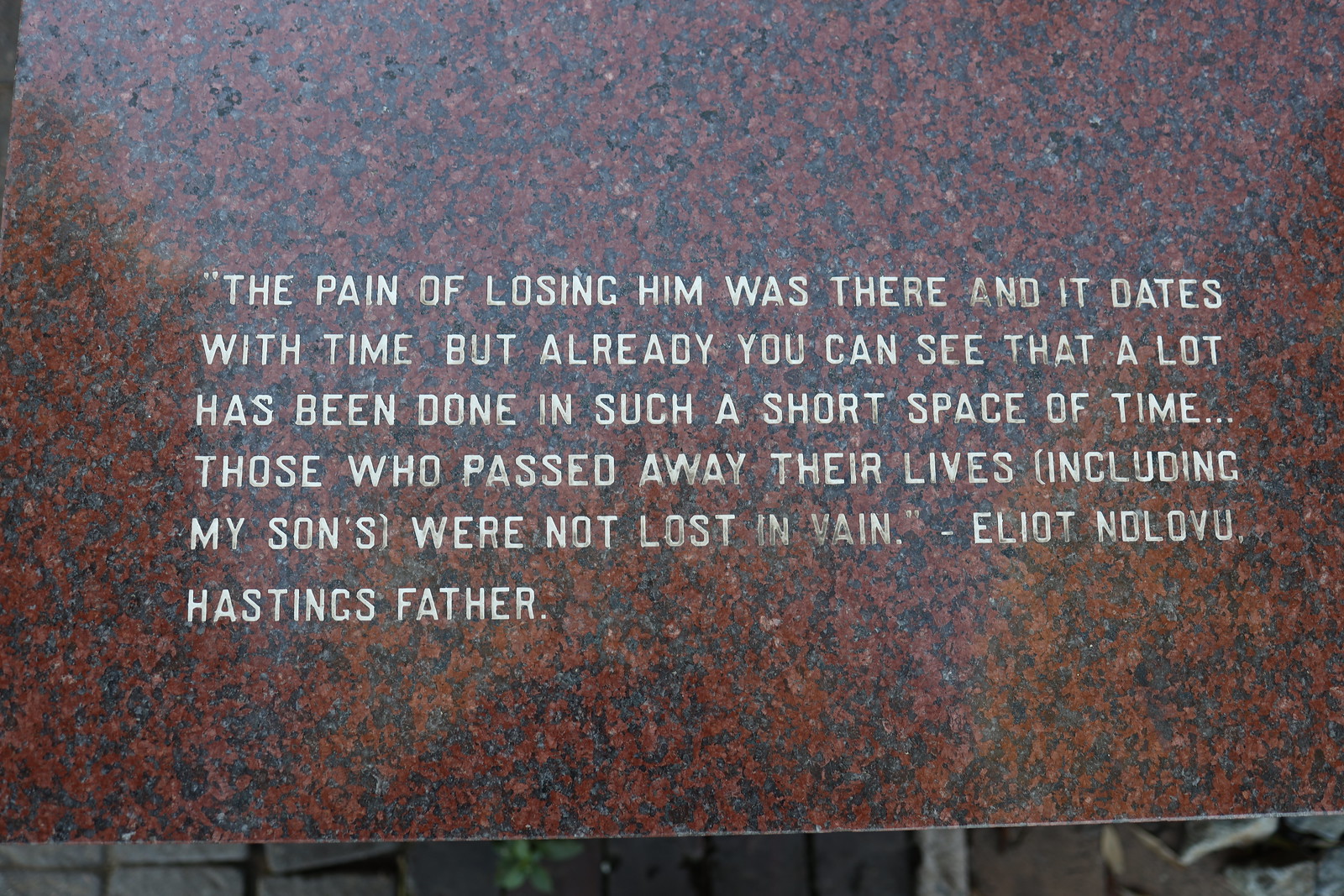The image captures a textured, dark charcoal gray tombstone or memorial plaque with a mottled surface. This central object occupies most of the frame, with a glimpse of what appears to be stone brick flooring at the bottom, suggesting an outdoor setting, possibly a graveyard. The plaque features an engraved quote in thin, white, all-capital letters, center-justified both vertically and horizontally. The inscription reads: "THE PAIN OF LOSING HIM WAS THERE, AND IT FADES WITH TIME. BUT ALREADY YOU CAN SEE THAT A LOT HAS BEEN DONE IN SUCH A SHORT SPACE OF TIME... THOSE WHO PASSED AWAY, THEIR LIVES, INCLUDING MY SON’S, WERE NOT LOST IN VAIN." The quote is attributed to Elliot Nolovu, Hastings' father. The colors in the image predominantly include shades of gray, green, white, brown, black, and tan.